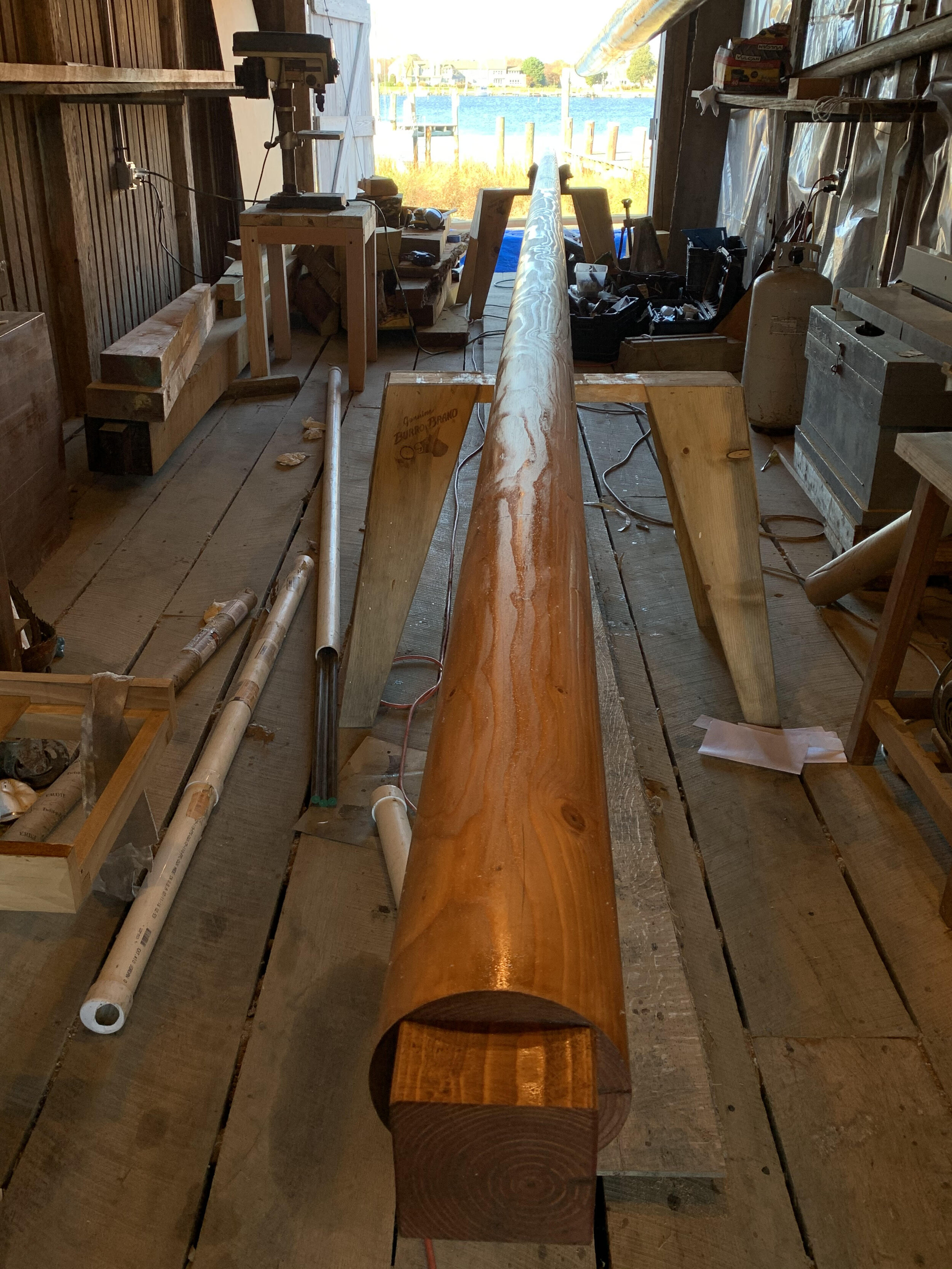This detailed image captures the interior of a rustic, open-air wooden workshop located in a long rectangular shed with aged wooden planks forming the floor. Dominating the center of the photograph is a meticulously smooth, varnished log bordered by two saw horses. The log’s rich, chocolate-brown finish suggests it's been carefully sanded and cared for, possibly using an adjacent wooden lathe or roller, also visible in the image.

To the left side of the space, a wooden wall houses an electrical outlet supplying power to a jigsaw situated on a worktable. Below, various tools and materials—including PVC pipes with steel bars, and a few boxes—are scattered on the floor.

On the right side, the light flooding in through an open, barn-style door at the end of the shed highlights additional items: a toolbox, a metal propane tank, and another worktable. Beyond the open door, glimpses of a large waterway flanked by piers and distant structures introduce a serene, waterfront setting into the workshop’s industrious atmosphere.

The wooden walls and exposed insulation give the building an old, time-worn character, enriched further by the assortment of tools that complete this snapshot of a bustling and well-used woodshop bathed in natural light.